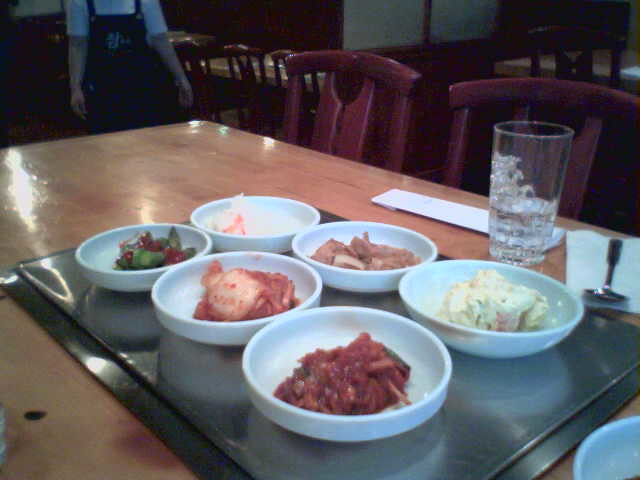In the image, a polished, sealant-covered wooden table shines under the restaurant lights. Placed upon the table is a metal tray holding six shallow, white bowls, each filled with a different type of food. Among the dishes, there's pasta with red sauce, some sort of meat, and various fruits. A glass of water with ice, a spoon, and napkins are also neatly arranged on the table. Two red wooden chairs are pushed into the table, ready for patrons. In the background, similar unoccupied tables and chairs can be seen, maintaining the restaurant's cohesive decor. On the top left, a person in an apron and a short-sleeved white t-shirt walks towards the table, their face out of frame.